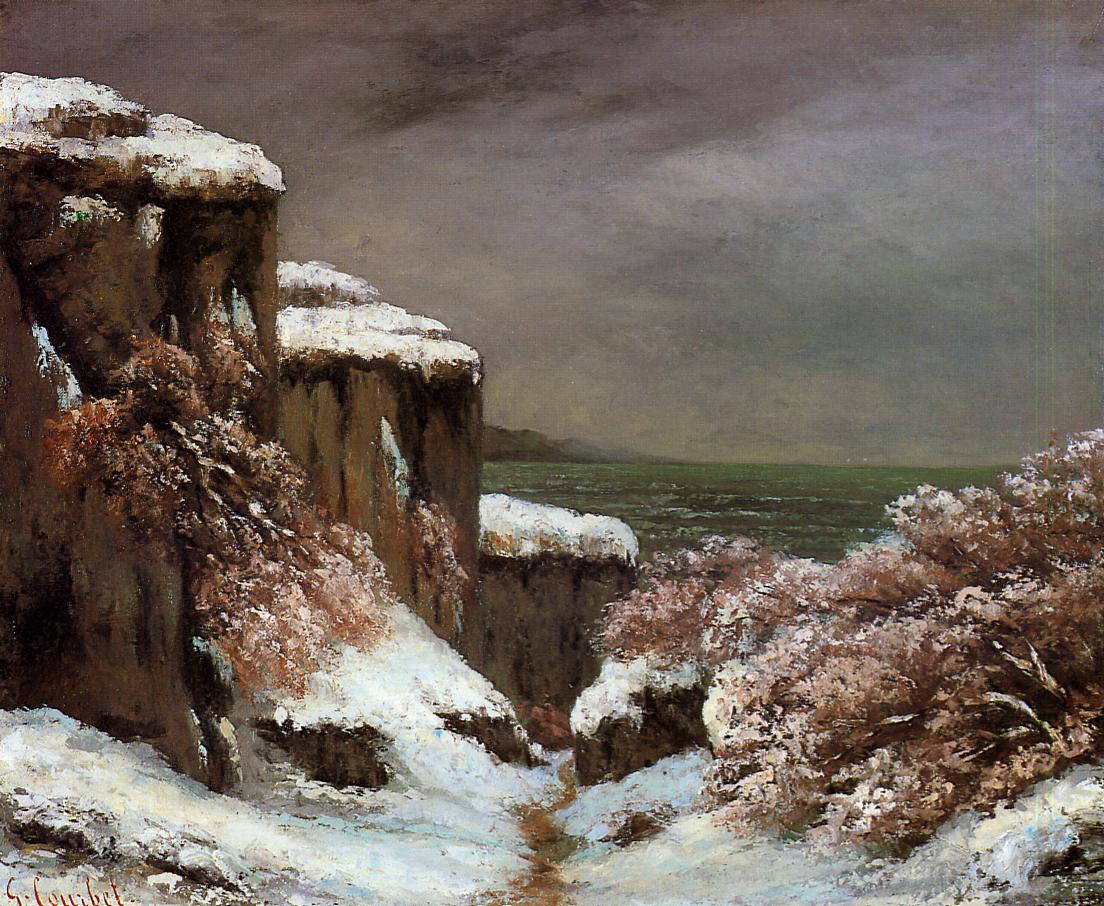The painting captures a snowy landscape with a prominent rock formation on the left side that resembles a large staircase, with snow-topped layers descending like steps. The tallest step is nearest to the left edge, followed by medium and shortest steps that lead towards the center-bottom of the frame. On the right side of the painting, there are bushes and some wild orangish plants, partially covered in snow, alongside a thin dirt path that weaves behind the rock formation. This path seems to extend from the bottom center of the image, potentially reaching down to a green-colored body of water that lies further in the background. Above the scene, the sky is overcast with gray, almost white hues. In addition to the main elements, a glimpse of distant hills and some scattered trees can also be observed. The artist's name appears faintly in the bottom left corner, though it is not fully legible.